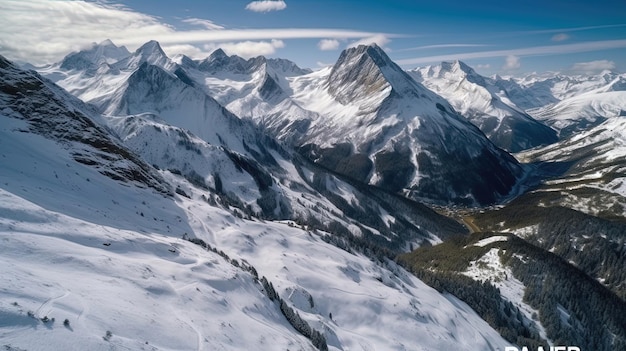This photograph captures a stunning, expansive mountain range under a clear blue sky with scattered, white clouds. The landscape-oriented image showcases numerous snow-capped peaks extending across the horizon. In the lower left part of the image, a hillside descends into a lush valley filled with greenery and trees. The valley, situated in the lower right quadrant, features interspersed patches of white snow amidst the green foliage, framed by the stony, towering mountains above. Shadows cast from the left highlight the mountainous terrain's relief and add depth to the scene. While there's a hint of text cropping at the photo's bottom edge, the main focus remains on the serene and majestic natural landscape, free from human presence or additional elements.